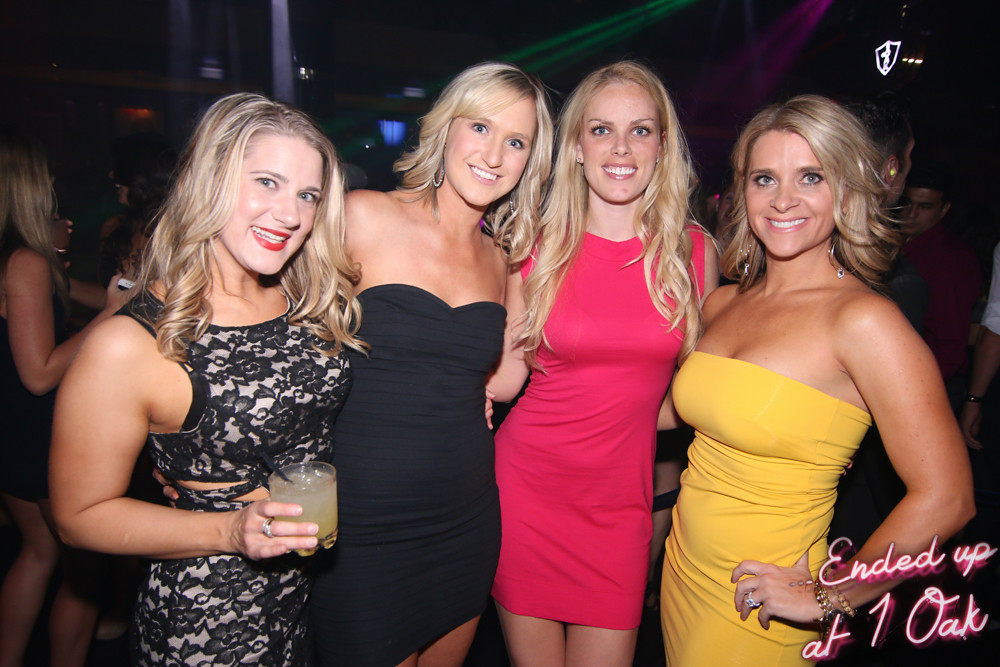The photograph features four blonde women standing together in a line with their arms around each other, all smiling brightly and showing their teeth. The setting appears to be a dimly lit club called One Oak, as indicated by the text in the bottom right corner. On the far left, the first woman wears a sleeveless black and white lace dress and holds a glass filled with a yellow liquid. She has long, middle-parted blonde hair and bright red lipstick. The second woman from the left wears a solid black tube top dress, tilting her head slightly to the right with her hair parting to the left. The third woman dons a pink sleeveless dress and has her hair parted on the left side. The woman on the far right wears a yellow tube top dress and has shorter hair parted on the left side. The background shows a dark club atmosphere with blurred figures and colored lights, enhancing the lively party setting.